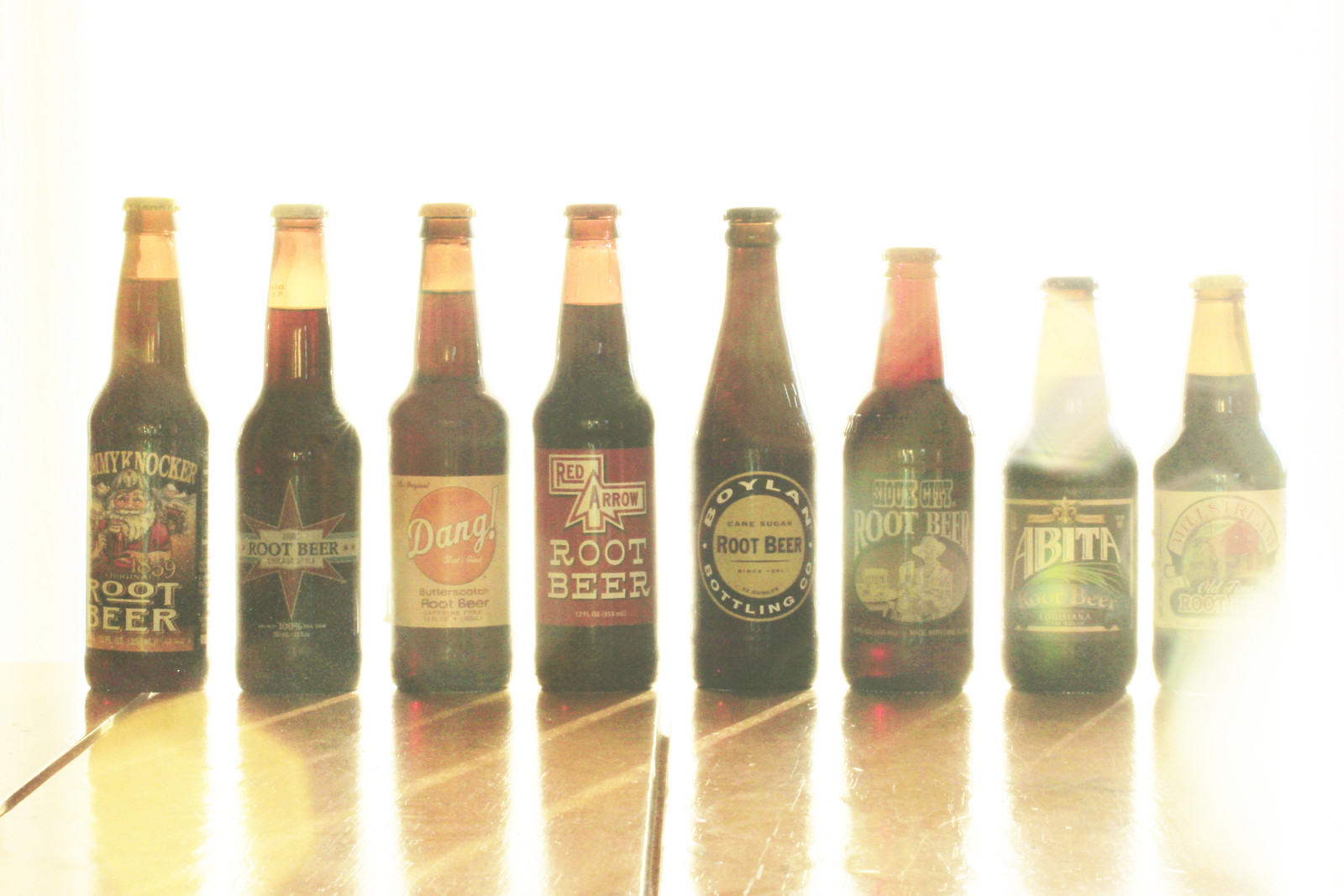The color photograph captures eight distinctive glass root beer bottles arranged in a line on what appears to be a wooden table. The image is heavily overexposed, causing the background to become a brilliant white with no discernible details, and similarly overexposing the front right corner where one bottle becomes indiscernible. Despite the overexposure, we can identify the following details: the bottles, each featuring a unique label and design, are positioned on a surface that shows dark brown grout lines suggesting ceramic tiles or a wooden table with visible spaces between the planks. The bottles vary in size and shape; the five on the left are taller with longer necks, while the three on the right are shorter. The first bottle's label shows an image of Santa and "Tommyknocker Root Beer." The second bottle displays a starburst with "root beer." The third has a yellow label with "dang!" The fourth bottle features a red arrow with "Red Arrow Root Beer." The fifth bottle is branded "Boylan Root Beer." The sixth bottle, labeled "Sioux City Root Beer," bears an image of a cowboy. The seventh bottle reads "Abita Root Beer" with a wave motif. The eighth bottle remains unreadable due to the intense lighting. This collection of variously labeled root beer bottles is framed against a blinding backdrop, highlighting the diversity of labels and designs even amidst the photograph's distortions.